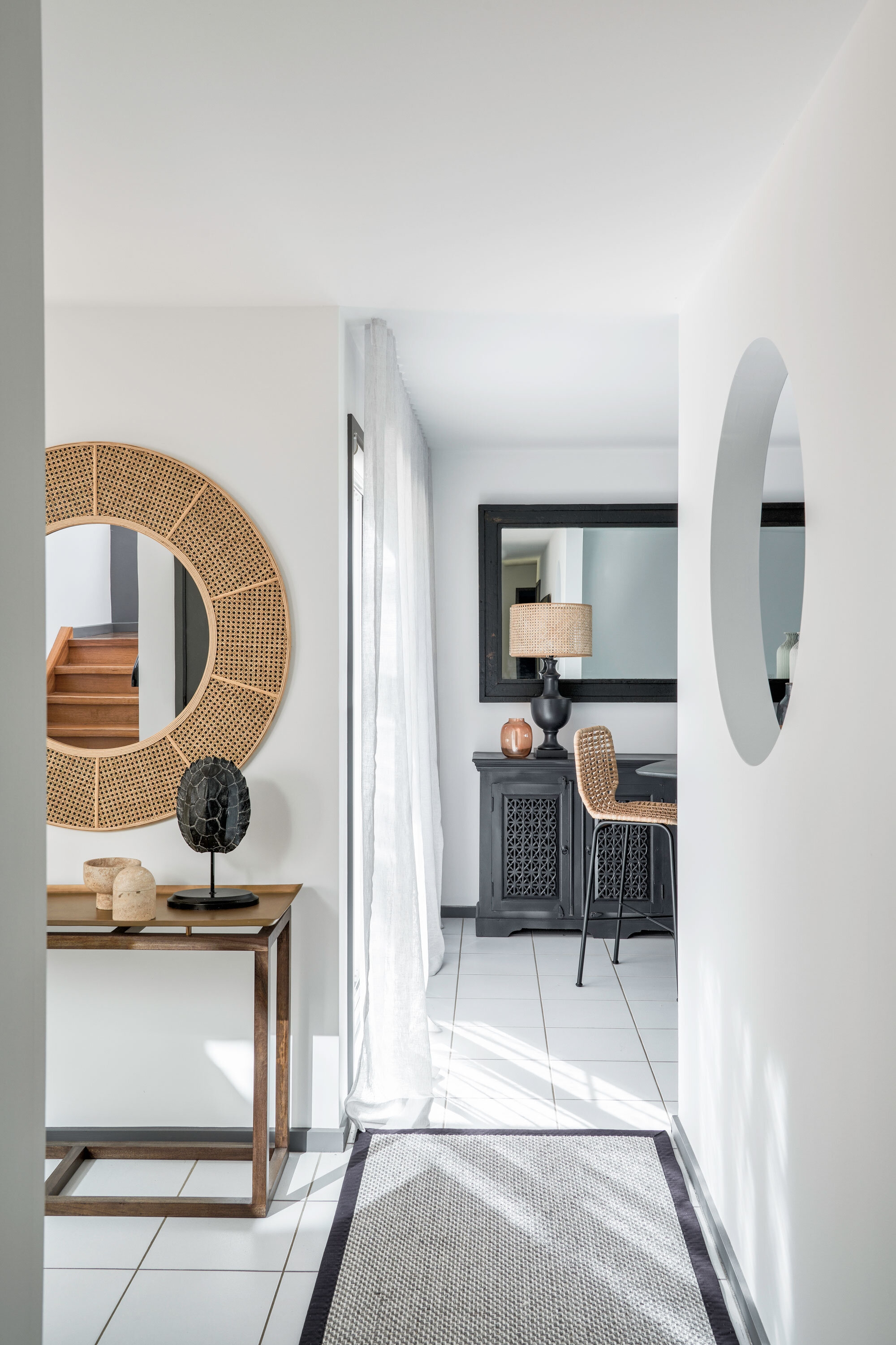This image captures the sophisticated and modern interior of a newly built house, likely taken from the foyer. The living area is framed by pristine white walls and a floor adorned with polished 12x12 white tiles with contrasting dark grout. A circular mirror with a stylish khaki woven frame is mounted on the left wall, paired with a matching decorative stand that holds various knick-knacks, including a tribal bowl and mask.

Directly in front of the view is a perfectly aligned runner leading towards white curtains covering what appears to be either a sliding glass door or an exterior door. A wall on the right side features a dramatic circular cut-out that offers a glimpse into an adjacent room, adding to the modern aesthetic. Additionally, the image captures a large black mirror on the opposite wall, below which sits a long bureau likely intended for dining room use.

In the mirror's reflection, one can discern a stairway leading to a second floor, suggesting that part of the space remains unseen. This thoughtful portal through the wall invites curiosity about the interconnected rooms and the overall architectural flow of the house. The combination of sleek design elements and thoughtful decorative touches makes this living space both functional and visually appealing.